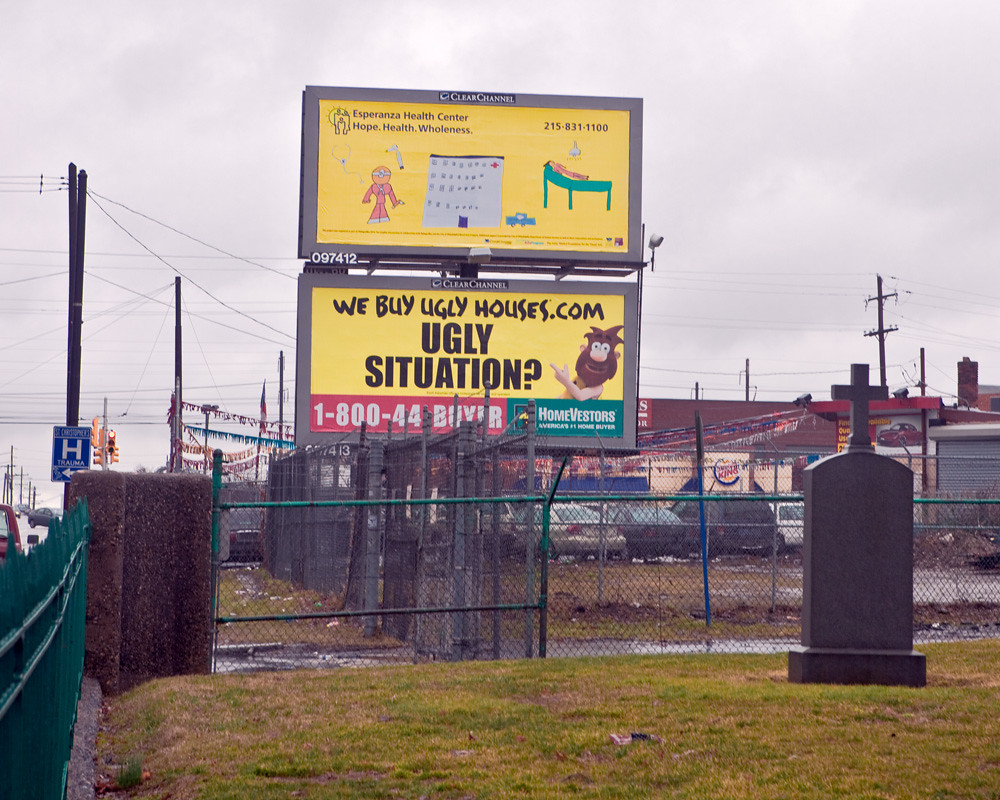The image features a vertically split billboard situated amidst a quaint town backdrop. The upper section of the billboard advertises Esperanza Health Center with the tagline "Hope, Health, Wholeness" set against a bright yellow background. This portion is adorned with charming, child-like drawings, including a doctor equipped with a stethoscope and various medical tools, a playful calendar, a car, and a person lying on a hospital bed, all contributing to a wholesome and inviting visual. Contact information for the health center is prominently displayed.

Beneath this is an ad for WeBuyUglyHouses.com, with the slogan "Ugly situation?" followed by their contact number. This part denotes Homevestors as "America's number one home buyer."

In the background, a Burger King and a car lot are visible. To the left, a street sign with "St. Christopher’s H" (indicating a hospital) points towards a trauma center. The entire scene is framed by a fence, and in the foreground, there is a tombstone, suggesting that the billboard is located near a cemetery. This intricate setting encapsulates a slice of life in a small town, blending elements of health, real estate, and daily life.